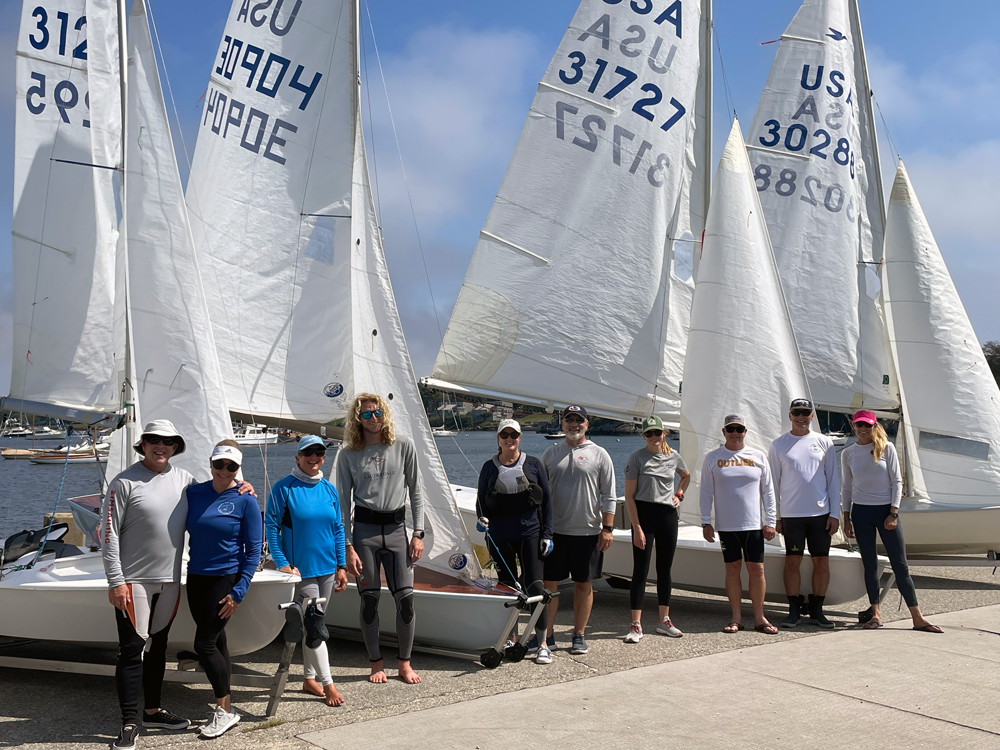This outdoor daytime photograph captures ten individuals, appearing to be five couples, each posing in front of a series of four small, white sailboats. Arranged in a line, the sailboats are positioned on land atop carrying carts, with the water of a bay or harbor and various larger boats visible in the background. Each sailboat, equipped with two white sails, features blue lettering that reads "USA" along with unique identifying numbers, suggesting they may have been used in a sailboat race. The people, who have Caucasian skin tones, are dressed in a mix of long-sleeved and short-sleeved shirts, shorts, and water pants; some are barefoot while others sport tennis shoes. The crews stand on a paved cement walkway, clearly identifiable as pairs, with the serene setting of a hill adorned with houses and a sky dotted with white clouds stretching out behind them.